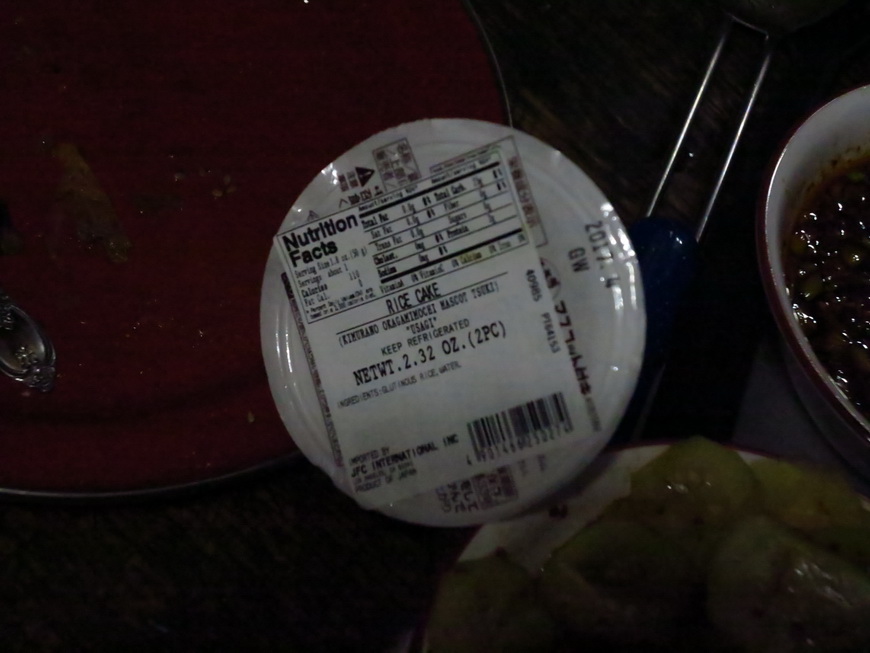The image captures a dimly lit scene centered around a rice cake label. The label prominently displays vital information including "Rice Cake," "Net Weight: 2.32 ounces," and "Two Pieces," along with detailed nutrition facts. Positioned in the lower right corner of the label is a barcode. This label is affixed to a white metal cap, below which a two-pronged silver handle extends from what appears to be a pot or dish. In the right section of the image, the edge of a bowl or mug filled with some liquid is discernible. Additionally, a brown circular object is visible in the bottom right corner of the frame. Most of the background remains engulfed in darkness, further highlighting the elements described.